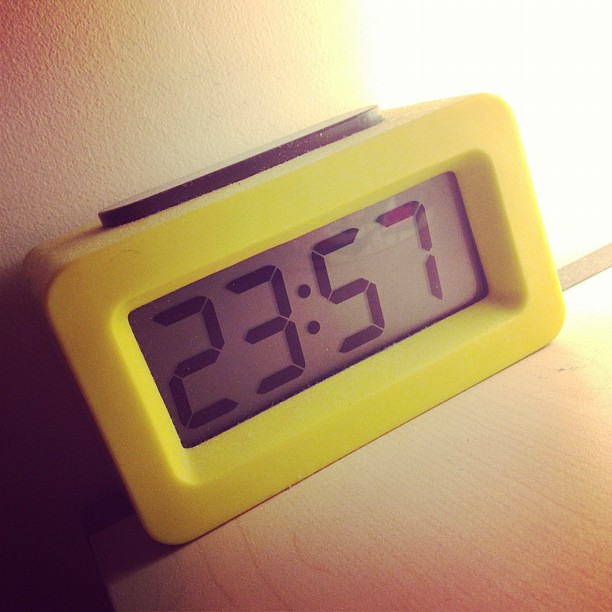In this photograph taken in a dimly lit room, a small, cube-shaped digital alarm clock commands attention from its spot on a wooden table. A bright, bedside table lamp casts a focused light from the top right-hand corner, illuminating the clock and highlighting its vibrant, thick plastic yellow frame. The clock's face is a soft grey with bold black digits displaying the time as 23:57. A raised black section, presumably a button, sits atop the clock, adding a tactile feature to its design. The overall atmosphere is cozy, suggesting a tranquil night-time setting.